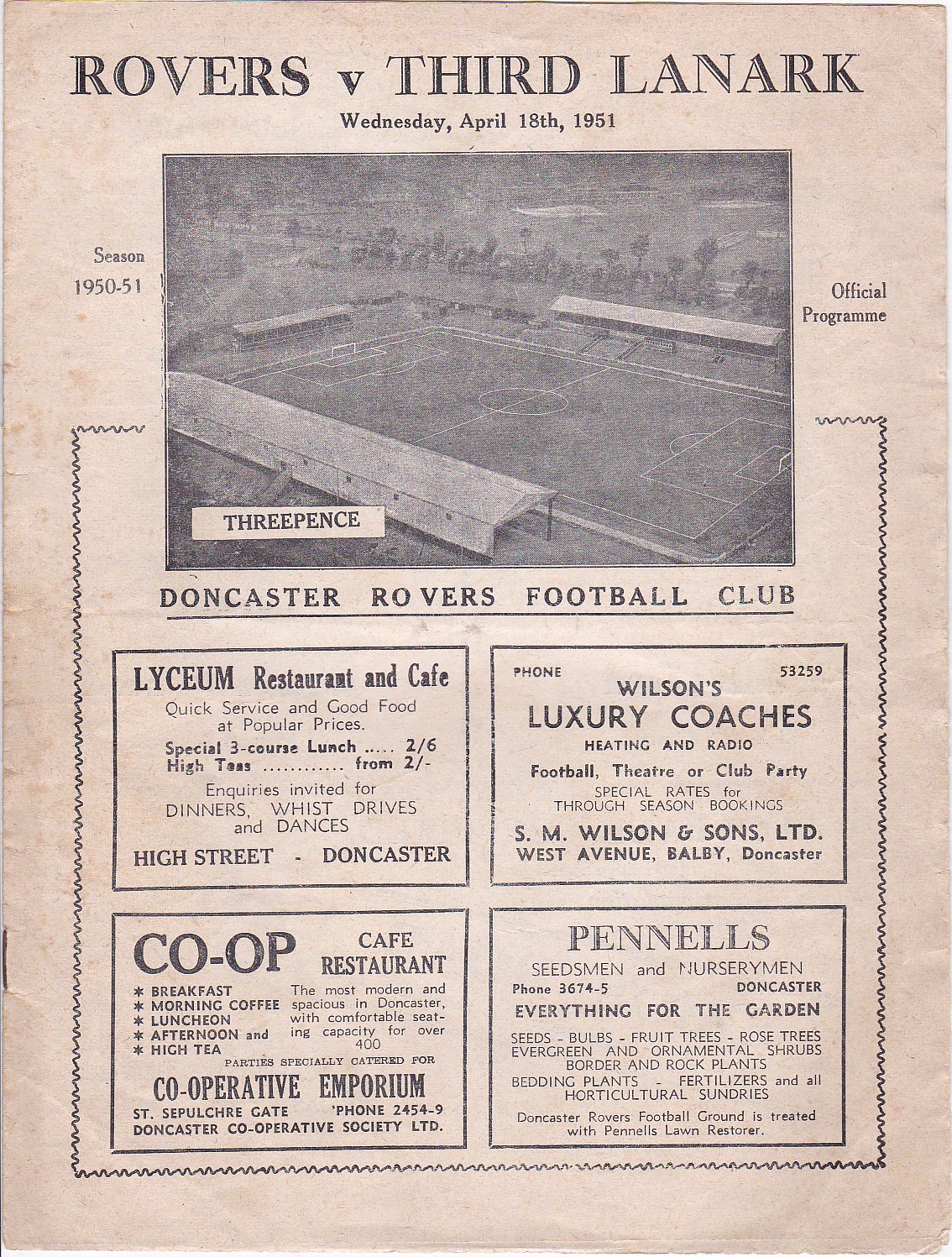This image depicts a discolored, vintage page from an old newspaper or magazine, showcasing an official program for a soccer match held on Wednesday, April 18, 1951, between the Rovers and 3rd Lanark. The page, marked by a dingy brown and black color scheme, features prominently displayed headlines: "Rovers v. 3rd Lanark," "Season 1950-51," and "Official Program." A staple is still affixed in the lower left-hand corner, indicative of its age.

The imagery on the page includes a faded, blurry photo of an empty soccer field with some covered seats visible on the sidelines. A small white rectangle within the picture states the price, "3 Pence." Below this photo, the text reads "Don Castor Rovers Football Club."

Underneath, there are four distinct advertisements, each enclosed in thin black outlines:

1. **Lyceum Restaurant and Cafe** - Promoting quick service, good food at popular prices, with special three-course lunches and high teas. They extend an invitation for inquiries about dinners, whist drives, and dances, located on High Street, Don Castor.

2. **Wilson's Luxury Coaches** - Highlighting luxury coaches equipped with heating and radio, available for football, theater, or club parties, and offering special season booking rates. The address is S.M. Wilson and Sons Limited, West Avenue, Balby, Don Castor.

3. **Co-op Cafe Restaurant** - Advertising extensive breakfast, morning coffee, luncheon, and afternoon and high tea services, boasting a spacious environment with comfortable seating for over 400 guests. They cater to parties specially, located at Cooperative Emporium, St. Sepulchre Gate, with a contact number of 2454-9, Don Castor Cooperative Society Limited.

4. **Pennell's Seedsmen and Nurserymen** - Offering a diverse range of gardening supplies, including seeds, bulbs, fruit trees, rose trees, evergreen and ornamental shrubs, bedding plants, fertilizers, and other horticultural sundries. They note that Don Castor Rovers Football Ground is treated with Pennell’s Lawn Restorer.

These advertisements celebrate and support the 1951 soccer match, contributing to a rich, historical tapestry of local commerce and community involvement.